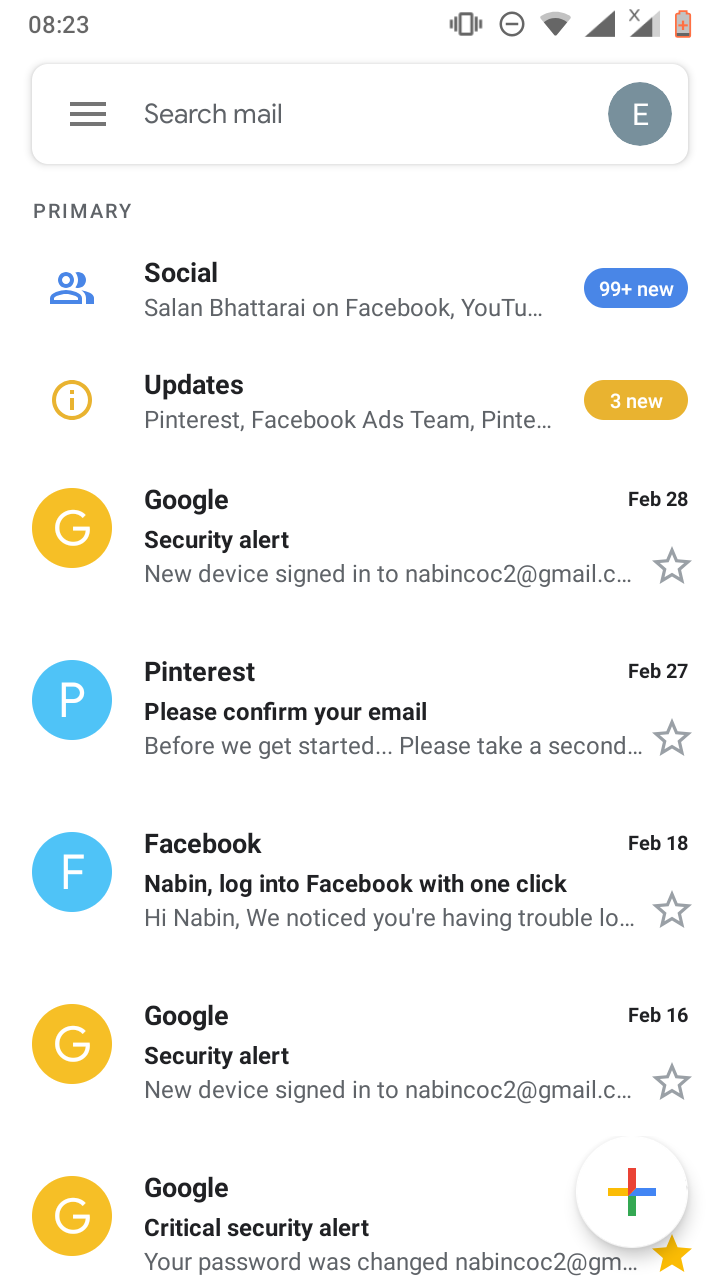The screenshot captures the display of a mobile phone's email application with a white background and black text. In the upper left corner, the time is shown as 08:23, indicating it is 8:23 in the morning. The status bar includes a vibrate icon represented by a circle with a line through it, Wi-Fi signal strength, cell signal strength, and another cell signal indicator, along with a nearly depleted battery icon.

Below the status bar, there is a search bar with three lines at the left, labeled "Search mail," indicating a feature to search through emails. Beneath the search bar is a gray circle with a white image inside; to the circle’s left, the word "Primary" is displayed.

A list of email categories follows, starting with "Social," highlighted in blue text, and featuring a blue circle with white text indicating "99+ new" messages. Below "Social," a yellow circle with an "I" in it denotes the "Updates" category, with messages ranging from Facebook, YouTube, and Pinterest notifications.

Further down, various notifications are listed: a yellow circle with a white "G" for Google-related updates, indicating a security issue or a new device login on February 28th, and similar entries for Pinterest on February 27th, Facebook, and multiple Google security updates.